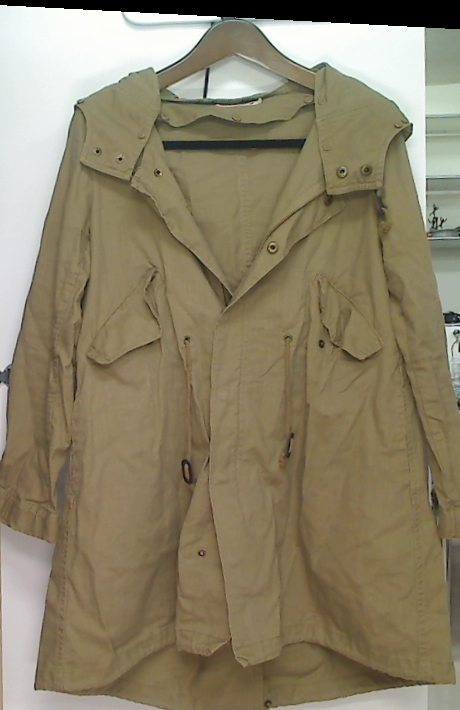This photograph, likely taken with a phone given its tall aspect ratio, showcases a khaki-colored raincoat prominently displayed on a sturdy wooden hanger against a white wall. The coat, which features a hood, is solid in color and has a sleek, slightly glossy finish hinting at weather-resistant material. It is adorned with black button-like snaps, with the female ends on the wearer's left and the male ends on the right, running down the front. There are also two snaps at the throat, allowing it to be fastened tightly around the neck. The interior of the coat is also brown, maintaining a uniform appearance. The front of the coat has two slanted pockets, one on each breast, and a drawstring at the waist, although there are no lower pockets visible. The coat appears to be of moderate length, extending just past the hips. In the background, a second white wall with three shelves is visible at the right edge of the image, with an indistinct item on the bottom shelf. Across the top of the image, an uneven black pixelated line runs from left to right, suggesting it may have been added digitally post-capture.